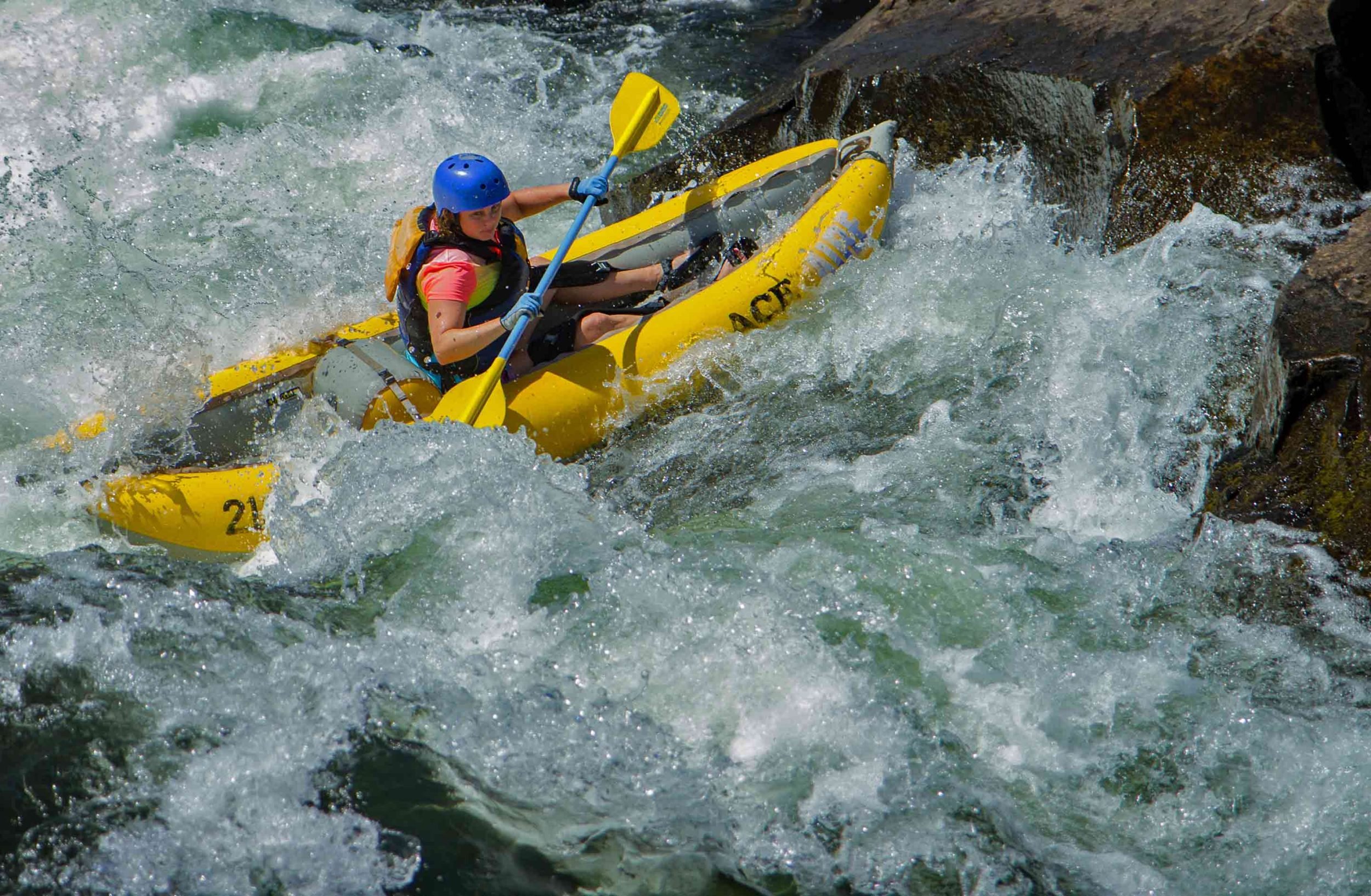In this vibrant and thrilling photograph, a woman is navigating a challenging whitewater rapid in an inflatable yellow kayak-canoe hybrid. She sports a short-sleeve pink and green outfit, covered by a blue life vest with a striking yellow section on the back, and a blue helmet for safety. Her hands are gripped firmly around a blue and yellow double-bladed paddle, perfect for maneuvering in the turbulent waters. The kayak bears the label "ace" and the number "21" on its side. 

As the woman paddles through the wild and clear blue-green water, she faces the intense whitewater head-on, with her kayak appearing slightly tilted and splashes of water surrounding her. The scene captures a moment of dynamic motion as she expertly navigates around treacherous brown rocks, her expression one of focused determination. She is outfitted with blue and black gloves, knee and thigh pads, and what appear to be water shoes or sandals, ensuring she is well-prepared for the adventure. The photograph, taken from a side view, freezes the action brilliantly, highlighting the frothing water and rocky terrain that make the rapid look both beautiful and dangerous, with the water thundering down at high speed.